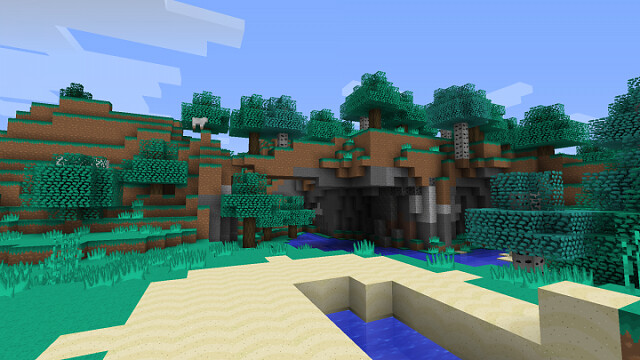The image appears to be a screenshot from the popular game Minecraft, showcasing a scenic landscape rendered in the game's characteristic blocky style. The scene is broad and detailed, featuring a variety of natural elements. In the foreground, there are numerous trees and bushes interspersed with patches of grass, while the background displays rolling hills and what appears to be the entrance to a cave. Prominently featured is a uniquely shaped sandy-colored oval area, partially visible with water contained within it, which might be a pool. This pool has a raised edge on one side, with the rest being level with the ground, suggesting some man-made or natural formation. Adding life to the image, a sheep can be seen standing atop one of the hills on the left side of the screenshot, contributing to the immersive, pastoral scene typical of Minecraft's creative environments.